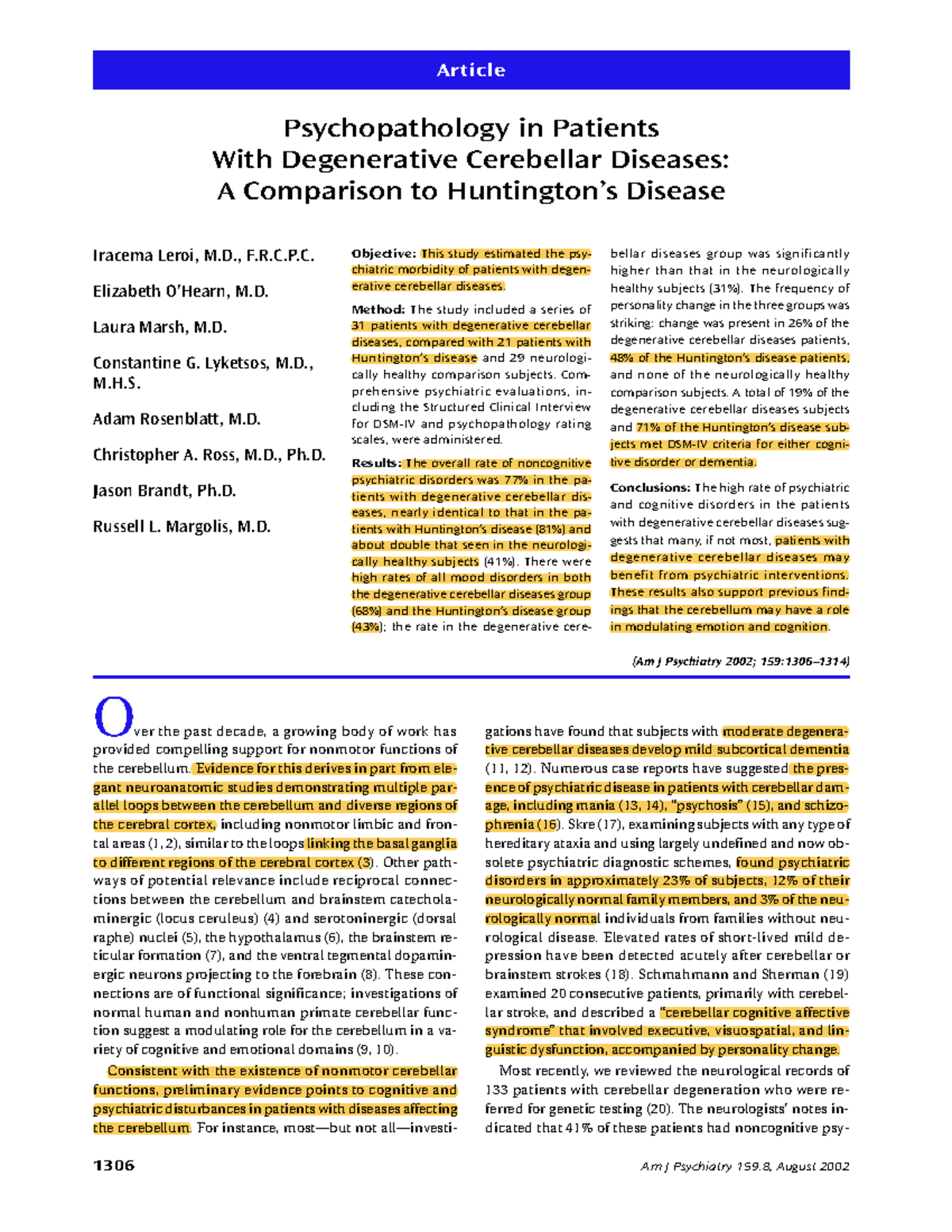The image features a detailed academic article layout.

At the top, within a blue header, the title "Article" is prominently displayed. Beneath this header, the article title "Psychopathology in Patients with Degenerative Cerebellar Diseases: A Comparison to Huntington's Disease" appears in bold black text.

The left side of the page lists the authors, presumably a group of doctors, all names printed in black text. On the right side, there is a section titled "Objective," which states: "This study estimated the psychiatric morbidity of patients with degenerative cerebellar diseases."

Certain texts in the article are highlighted in an orange-like color for emphasis. Below the "Objective" section is the "Method" section, which details the study's design. It indicates that the study included a series of 31 patients with degenerative cerebellar diseases, 21 patients with Huntington's disease, and 29 neurologically healthy comparison subjects. The study employed comprehensive psychiatric evaluations, including the Structured Clinical Interview for DSM-IV and various psychopathology rating scales.

Further down the page, a "Conclusion" section is briefly mentioned. Beneath this section, a blue bar separates this article from another piece titled "Over the past decade, a growing body of work has provided compelling support for non-motor functions of the cerebellum." This is followed by several paragraphs of related text.